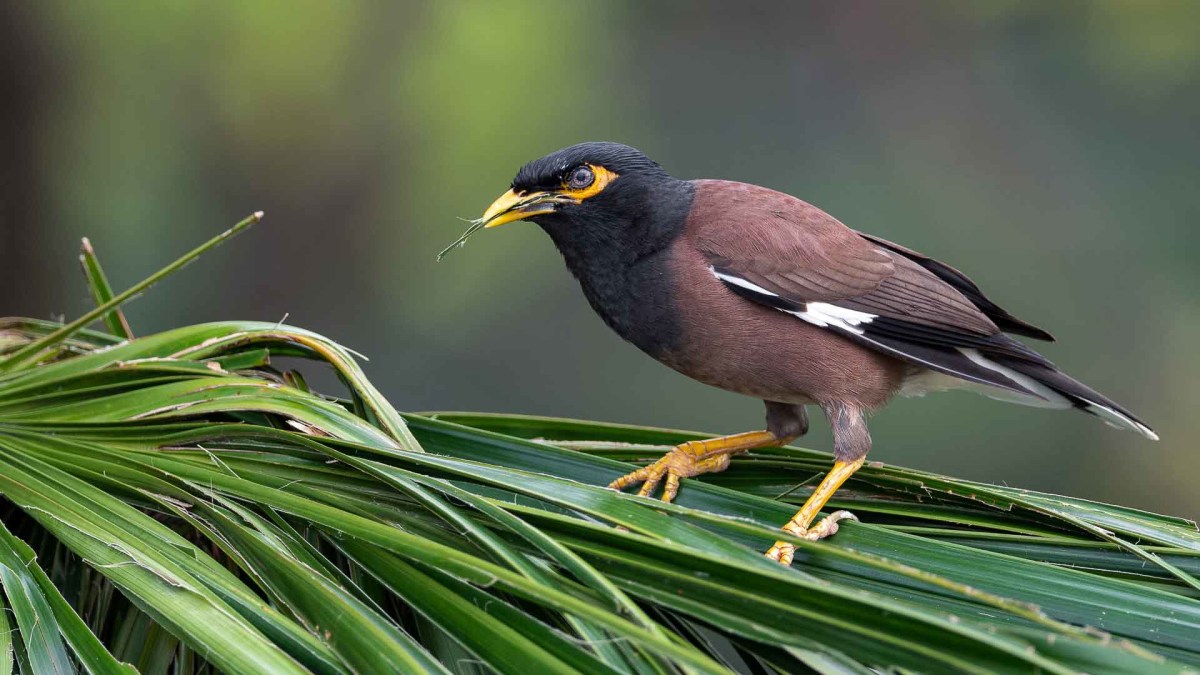In this macro-style photograph, an Indian Myna bird is prominently featured. The background is artistically blurred, highlighting the bird amid a backdrop likely consisting of leaves and plants. The bird's distinctive features are well-captured: a black head and chest plumage transitioning into reddish-brown in the middle, while its wings and tail exhibit striking black and white feathers. Its limbs are yellow, and its beak, along with the pattern around its eyes, display a gold-like yellow hue. Interesting details such as the dark gray of the bird's eyes and the complete black pupil stand out. The bird appears to be engaged in nest-building, as evidenced by the piece of plant material—possibly a palm frond—clutched in its beak. It is perched on a tangled mass of ferns or leaves, with its claws gripping the foliage firmly. The Indian Myna seems poised, perhaps ready to take flight, as it gazes directly into the camera lens.